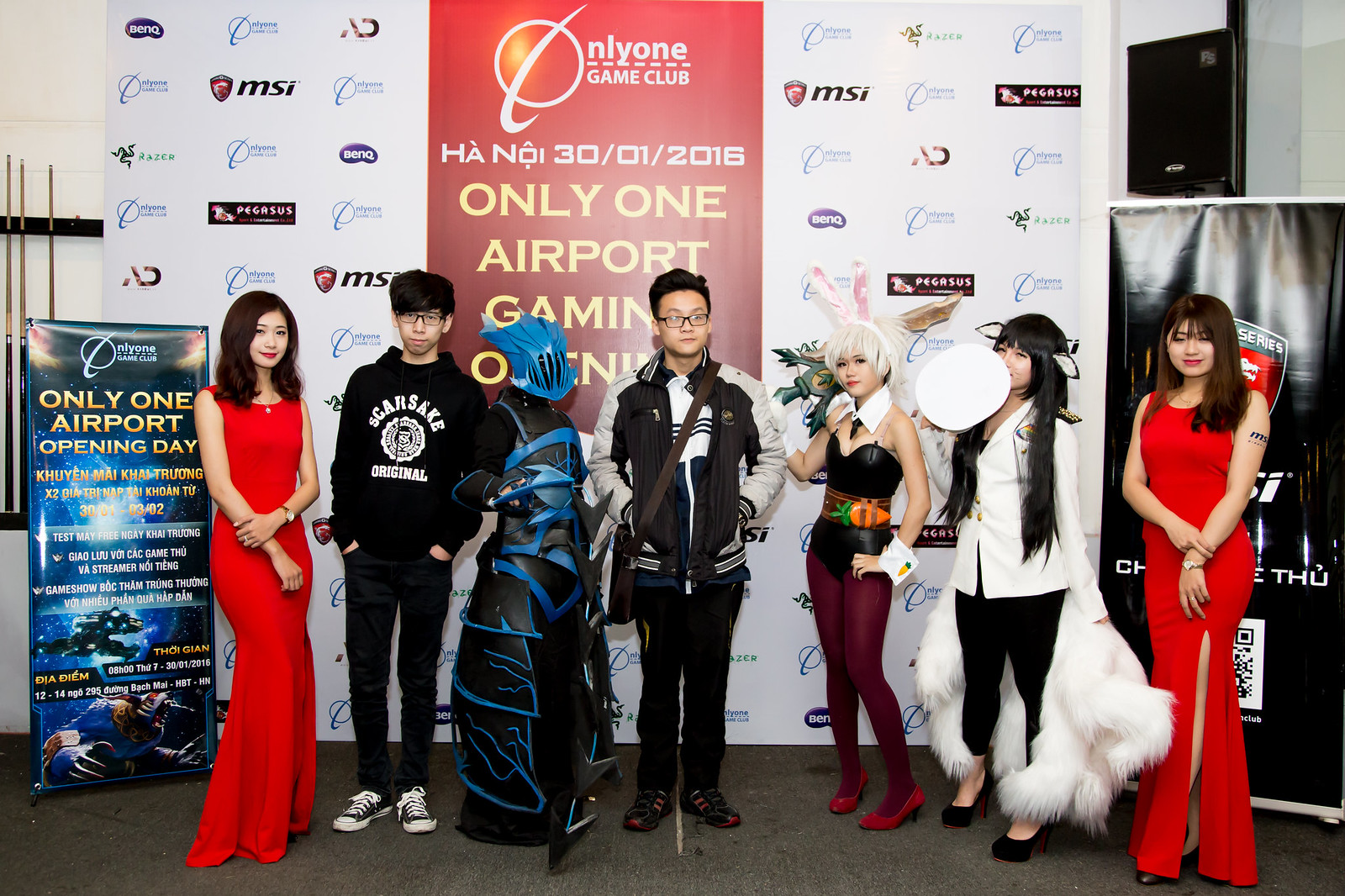In this image, seven young Asian individuals stand in a row, posing for a photograph on a carpeted floor. The two young ladies on the left and right are dressed in identical long red dresses, with the girl on the right featuring a temporary tattoo on her left arm that reads "MSI," matching the computer parts brand. Between them are five people, consisting of two young men and three young women, dressed in cosplay costumes likely representing characters from video games or anime.

The scene appears to be indoors, with various signs and logos visible on either side of the backdrop behind them. Prominently displayed in the center, the backdrop features a mix of colors including red, gray, black, tan, white, blue, green, and orange. It showcases the logos of sponsors such as MSI, the Bank, BenQ, and Pegasus, alongside "Only One Game Club." The text on the backdrop reads, "Only One Game Club, Hanoi, 30-01-2016, Only One Gaming Opening," indicating that the photograph was taken during the opening day of a game club event.